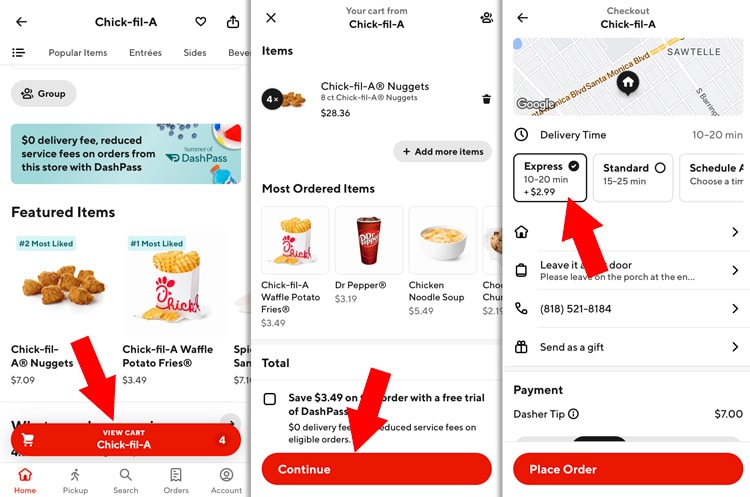The image comprises three sequential smartphone screenshots demonstrating the process of placing a delivery order from Chick-fil-A. Each screenshot has a white background, aligning them visually.

1. **Screenshot 1 (Left):** 
   - **Header:** The Chick-fil-A logo is at the top.
   - **Menu Categories:** Visible categories include Popular Items, Entrees, Sides, and the partially visible Beverages category. 
   - **Grouping Option:** To categorize items, a small gray rectangle labeled “Group” is present.
   - **Promotional Banner:** Below this, a light blue banner with dark blue text offers a zero delivery fee and reduced service fees with DashPass. 
   - **Featured Items:** Featured items section follows, showcasing Chick-fil-A Nuggets priced at $7.09, alongside an image of Chick-fil-A Waffle Potato Fries in a branded white container. 
   - **Action Button:** At the bottom, a red rectangle with rounded edges and white text reading “View Cart Chick-fil-A,” emphasized by a large red arrow.

2. **Screenshot 2 (Middle):**
   - **Order Details:** Displays an order summary at the top with Chick-fil-A Nuggets, four portions totaling $28.36.
   - **Most Ordered Items:** Lists popular items like Chick-fil-A Waffle Potato Fries, Dr. Pepper (represented by a tall takeaway cup with the logo), Chicken Noodle Soup (shown in a white bowl), and a partial image of Chocolate Chunk Cookies.
   - **Action Prompt:** Reiterates the red “View Cart Chick-fil-A” button and red arrow.

3. **Screenshot 3 (Right):**
   - **Order Finalization:** 
      - **Location:** A small Google Map thumbnail at the top indicates the restaurant's location.
      - **Delivery Options:** Shows the selected “Express Delivery” option, promising delivery in 10-20 minutes for an additional $2.99, indicated by a red arrow.
      - **Details and Preferences:** Options to “Leave at door,” along with fields to enter phone number, send as a gift, and payment details appear next.
      - **Dasher Tip:** Section for tipping the delivery person, with a suggested amount of $7.
      - **Place Order:** Finishes with a red “Place Order” button at the bottom.

These images collectively guide the user step-by-step through the Chick-fil-A delivery order process, emphasizing key actions with vivid annotations for clarity.